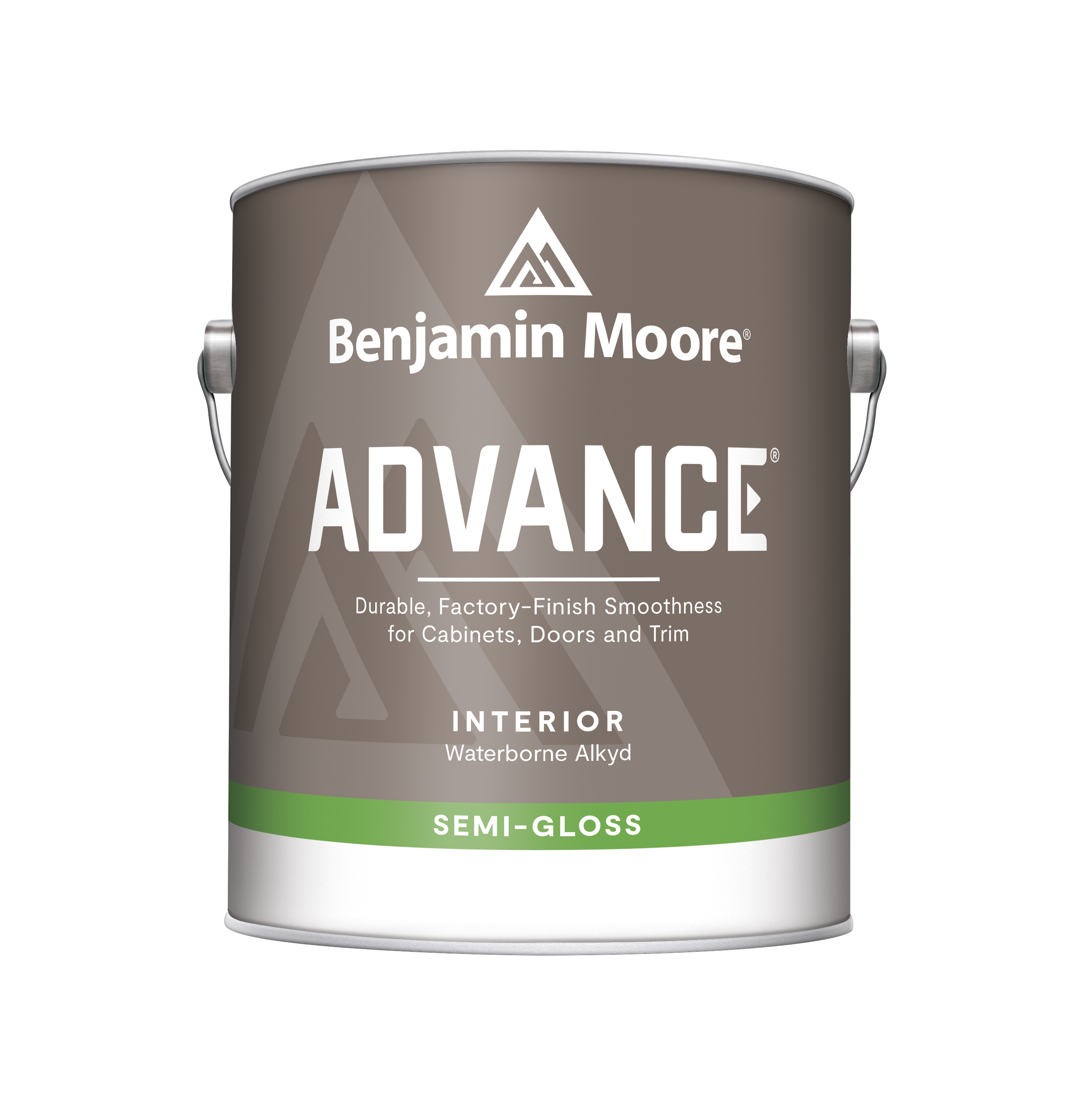The image depicts a can of Benjamin Moore paint set against a white background. The paint can is primarily gray with a green stripe across the middle, indicating it is a semi-gloss finish. Below the green stripe, there is a silvery base. The can features a triangle logo with an 'M' in the center, representing the Benjamin Moore brand. At the top, in white text, it reads "BENJAMIN MOORE," and below that in bold capital letters is "ADVANCED." The description on the can states "Durable factory finish smoothness for cabinets, doors, and trim." The can also has a silver handle with knobs attaching it to the sides.